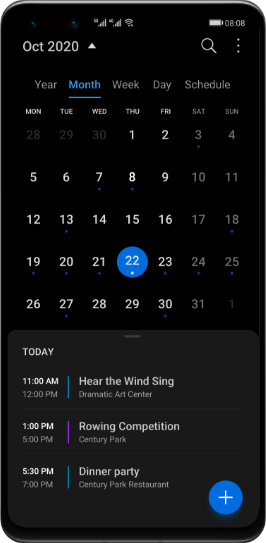The image depicts a digital interface that appears to be a detailed calendar or scheduling application. In the upper right corner, various icons are displayed, indicating signal strength with two status bars, WiFi connectivity, and a fully charged battery. The time is shown as 8:08 PM.

Directly below is the date section, stating October 2020, accompanied by an upward arrow. On the right-hand side, there are a magnifying glass icon and three vertical dots, suggesting search and more options.

The calendar view features different text colors and styles: the year is displayed in gray, the month in blue and underlined, and the labels for weekdays and "schedule" are in gray. Days of the week from Monday to Thursday are in white, while Saturday and Sunday are in gray. Corresponding day numbers are also shown in these colors.

Specific dates have notable annotations:
- Blue dots appear on the 3rd, 7th, 8th, 13th, 18th, 19th, 20th, 21st, 23rd, 24th, 25th, 27th, and 30th.
- The 22nd is highlighted in blue with a white dot.

A grayscale section below the calendar outlines various events for the day, such as:
- "Today, 11:00: 'with the wind sing'"
- "12:00: dramatic art center"
- "1:00: rolling competition"
- "5:00: Century Park"
- "5:30: dinner party"
- "7:00: Century Park restaurant"

At the bottom right corner, there is a blue circle containing a white plus sign, likely for adding new events or tasks.

This comprehensive layout provides a thorough overview of the user's schedule and relevant options for navigation and modifications.